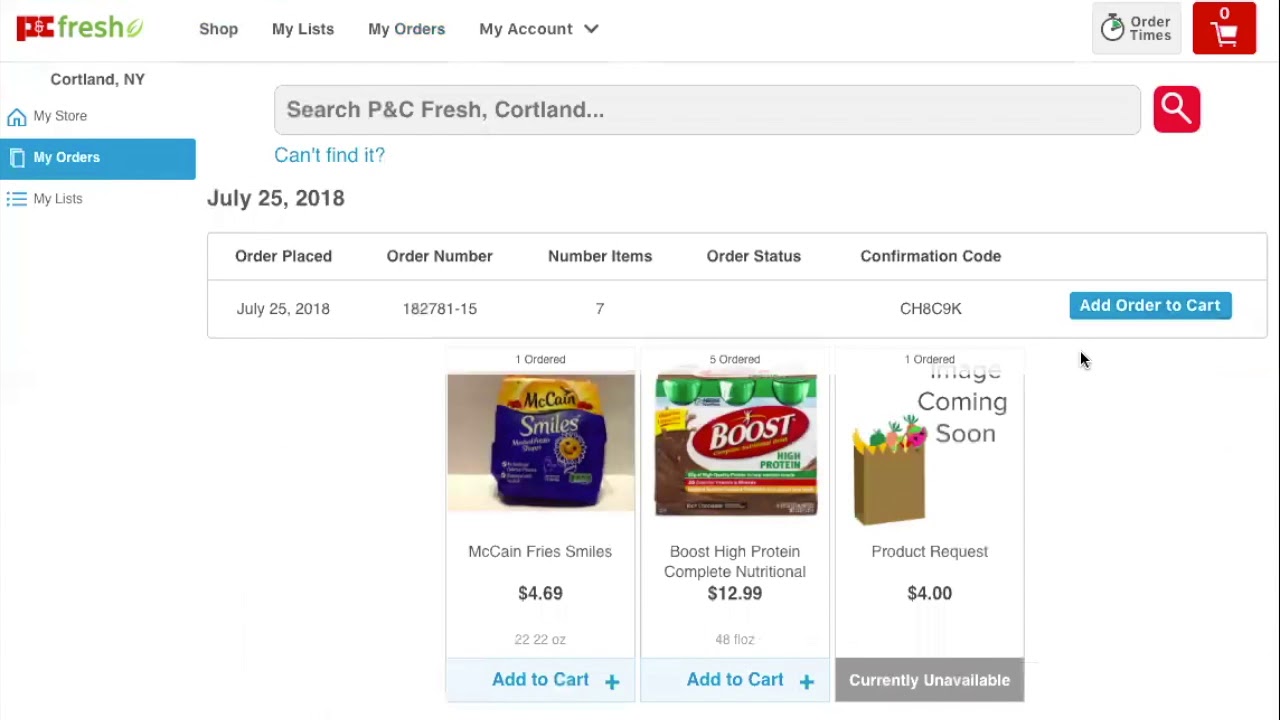The image depicts an online grocery delivery interface, predominantly colored in white with various text and icons in different colors.

**Top Navigation:**
- **Top Left Corner:** The word "Fresh" is prominently displayed in green lettering. Adjacent to it is a horizontal menu with the options: "Shop," "My List," "My Orders," and "My Account." There is a drop-down menu available next to "My Account."
- **Order Times and Cart:** Towards the right, there’s a "Order Times" indicator followed by a "0 Empty Shopping Cart" icon.

**Location and Search:**
- **Location:** The location "Cortland, New York" is highlighted and set for "My Orders." The menu here includes additional options like "My Store" and "My List," with "My Orders" currently selected.
- **Search Bar:** A long search bar labeled "Search PNC Fresh Cortland" is present, with a magnifying glass icon next to it.

**Main Section:**
- **Can't Find It:** Below the search bar, the words "Can't Find It?" are shown.
- **Date:** The date displayed is "July 25th, 2018."
- **Categories:** A horizontal row categorizing orders, labeled from left to right as "Order Place," "Order Menu," "Order Number," "Number Items," "Order Status," and "Confirmation Code."

**Detailed Order Information:**
- **Order Place:** Lists a date.
- **Order Number:** Shown below the date.
- **Number Items:** Displays the count of items in the order.
- **Order Status:** Currently empty.
- **Confirmation Code:** Presented on its own bar.
- **Add Order to Cart:** There’s an option to "Add Order to Cart" next to the order details.

**Product Images and Details:**
- **McCain's Smiles Fries:** A bag of frozen fries in smiley face designs, in a yellow and blue package, priced at $4.69 with an option to add to the cart.
- **Boost Protein Drinks:** A pack of six pre-mixed Boost high-protein nutritional drinks. The packaging features white lettering on a red background, with green bottle tops, priced at $12.99.
- **Image Placeholder:** A generic image placeholder that says "Image Coming Soon" with a basic illustration of a brown grocery bag, labeled as a "Product Request" priced at $4.00.

Each product includes detailed descriptions and pricing, intended for easy online shopping and ordering.